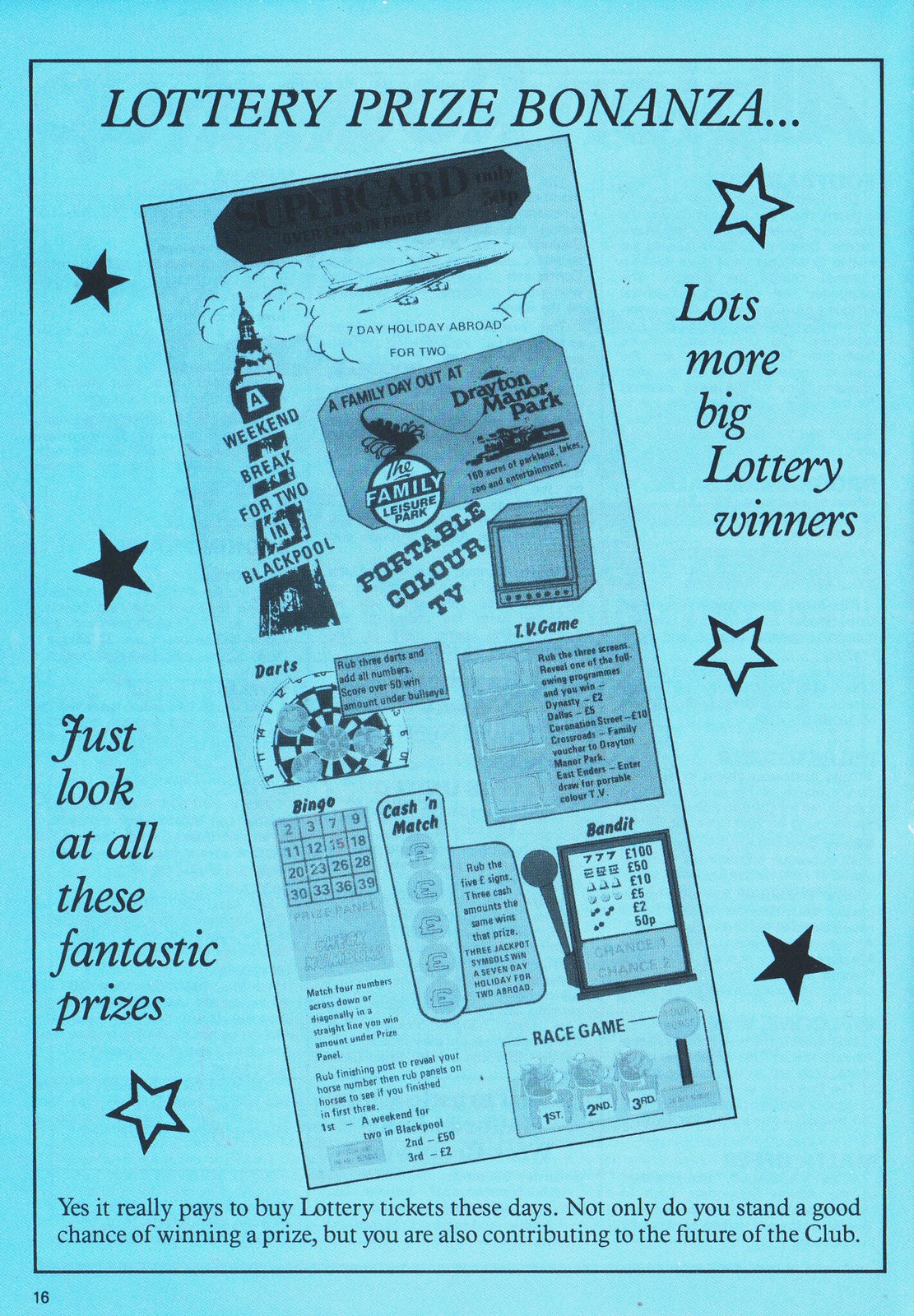The image displays a flyer advertisement on a light blue rectangular background with a black outline. At the top, it prominently reads "Lottery Prize Bonanza…" in bold black ink. Stars of different colors adorn the background—some are fully black, while others are outlined in black with white interiors.

On the left side, the text exclaims, "Just Look At All These Fantastic Prizes," accompanied by two stars. On the right side, it promises, "Lots More Big Lottery Winners," with another star beside it.

In the middle, a black outlined rectangle showcases several enticing prizes. These include visuals of an airplane with the text, "Seven-day holiday abroad for two," an old-school portable color TV, a weekend break for two in Blackpool illustrated by a high tower, a dartboard, a bingo number sheet, and a slot machine captioned "Match Bandit."

At the bottom of the flyer, it concludes with, "Yes, it really pays to buy lottery tickets these days. Not only do you stand a good chance of winning a prize, but you are also contributing to the future of the club," written in small black print.